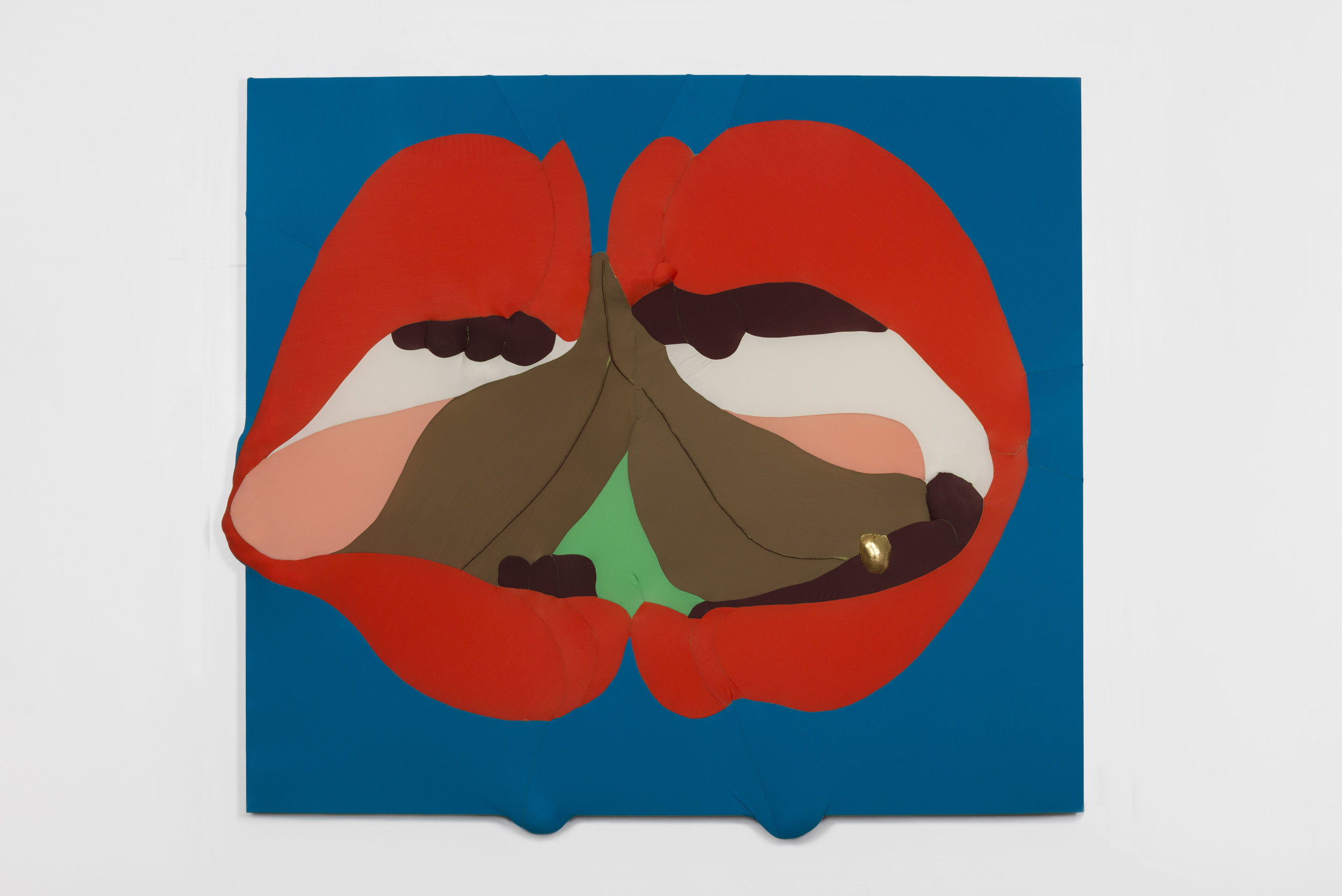The image is set against a light gray background featuring a blue square at its center, which frames the main subject. This central piece is a vibrant and abstract painting with multi-colored elements. Dominating the scene are two red, lip-like shapes that seem to be facing each other. Emerging from these red forms are brown and black protrusions, resembling teeth or perhaps eyelashes, adding a textured contrast. Flanking these are light pink structures on the left and right, evocative of tongues or possibly parts of an eye.

Central to the composition are light brown, tongue-like structures that originate at the top of the red shapes and extend downward, splitting into two symmetrical paths. Below this focal area of interaction lies a green section, which could be interpreted as a nose or another ambiguous feature.

The overall palette includes dark blue, red, black, white, beige, dark brown, and green, contributing to the modern art feel of the piece. The myriad of interpretations suggests an almost surreal quality, depicting either an emotive interaction between two mouths or an abstract facial composition.